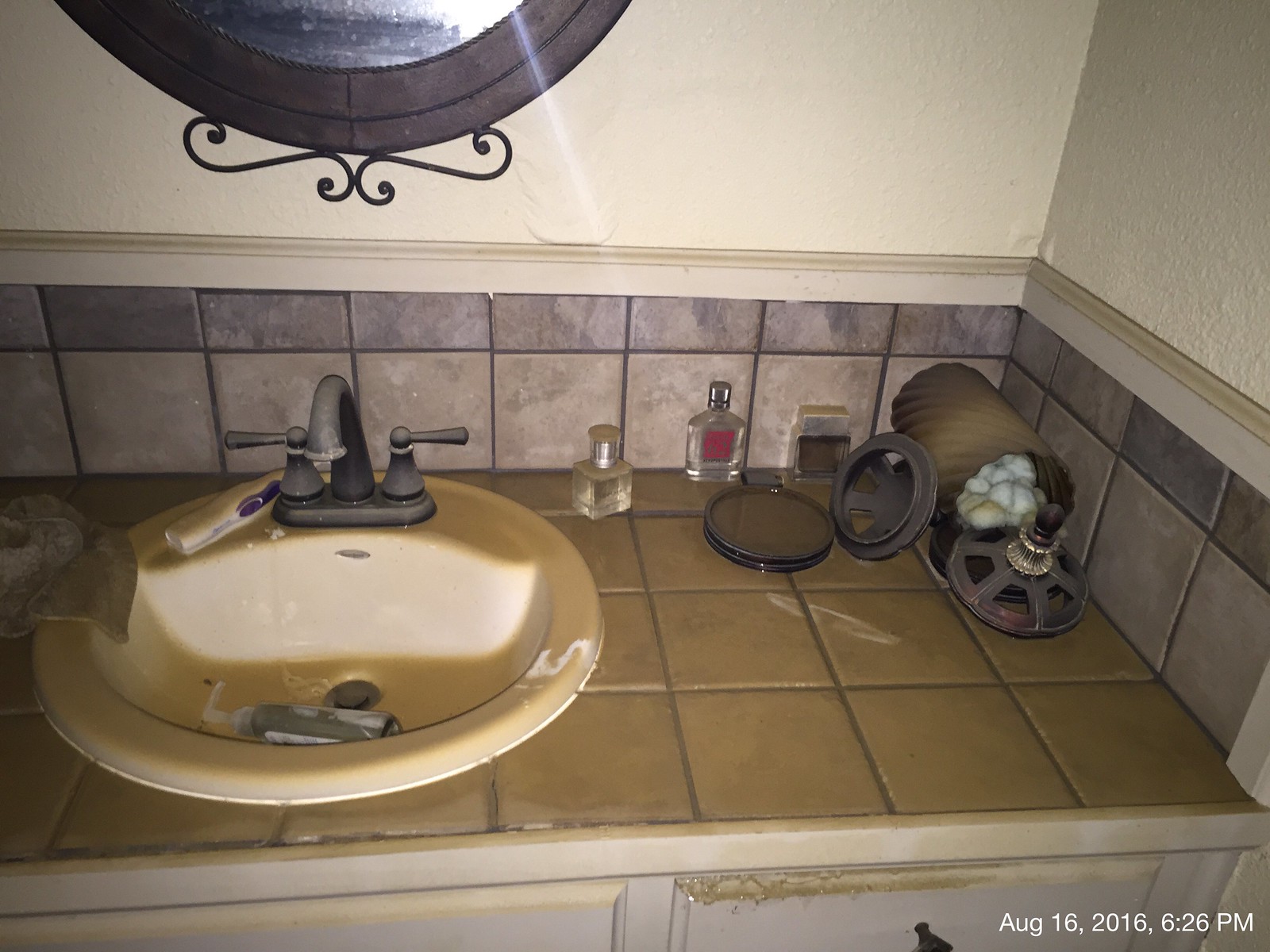This photo, marked with a timestamp of August 16th, 2016, at 6:26 PM in the bottom right corner, showcases a bathroom countertop under dim lighting conditions with a slight hint of brighter light entering the scene. The countertop is covered in brown tiles, complemented by a backsplash of smaller gray tiles, adding a contrast to the design. Above the backsplash, there is a white wooden ledge, leading up to a drywall wall painted white.

Centrally positioned above the bathroom sink is a black-framed mirror adorned with a decorative metal swirl beneath it. The sink itself is a unique orange color and is equipped with a single faucet. A pump-style soap dispenser has toppled into the sink, lying on its side. Next to the fallen soap dispenser, a purple and white toothbrush rests beside the faucet, adding a touch of personal detail to the scene.